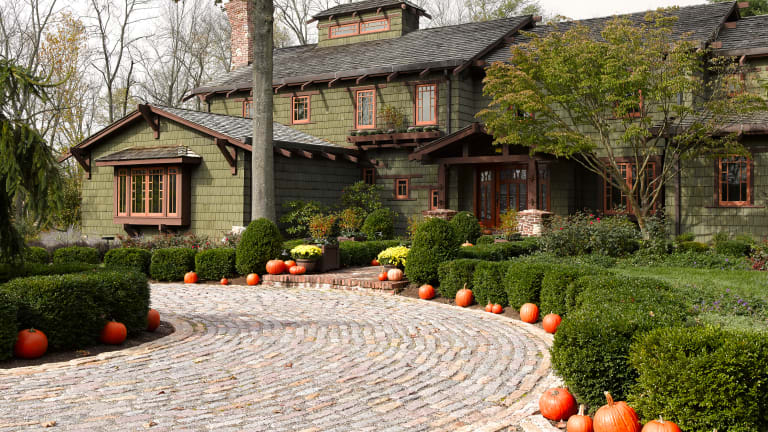This detailed image depicts a large, almost mansion-like green house with a mix of dark green shingles and siding, complemented by brown trim and windowsills. The roofing is a dark gray, sloped style with brick chimneys visible on the left-hand side. The structure spans two to three stories, with a smaller, third-story room noticeable at the top. 

The front yard is beautifully landscaped with manicured green shrubs and bushes surrounding the house, alongside a circular stone roundabout driveway and a red brick walkway leading up to the brown front door, which features a glass design. The overall ambiance suggests it is Halloween time, as the property is dotted with numerous pumpkins.

In the background, the sky is overcast, casting a white-gray hue, and the trees exhibit a mix of barren branches and some with yellowing leaves, particularly on the far left. Additionally, there is a noticeable contrast between the tall, lanky trees and the compact green bushes closer to the house. Overall, the home and its surroundings are impeccably well-maintained, with an evident Halloween theme represented by the abundance of pumpkins scattered throughout the yard and around the bushes.